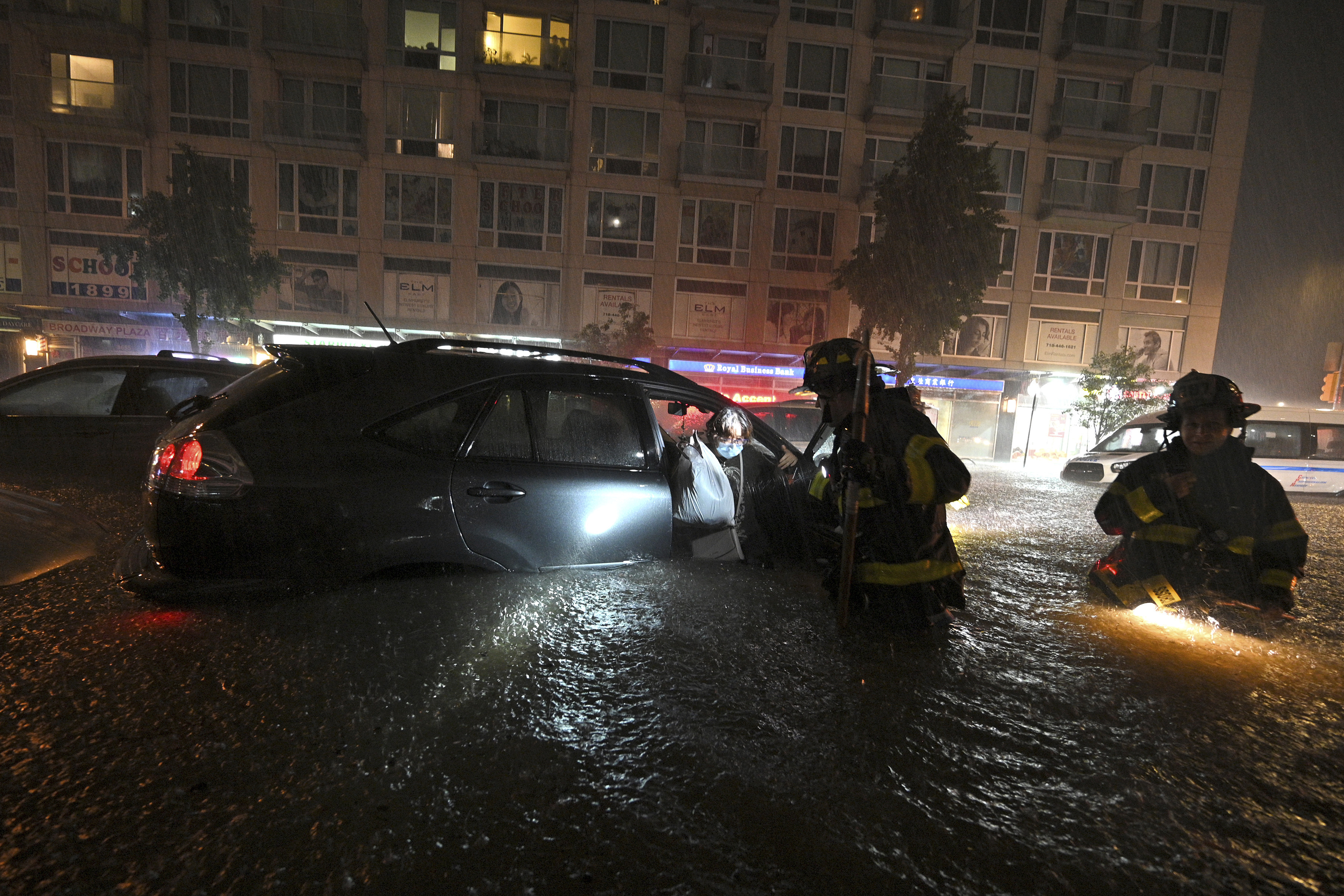The image depicts a vivid and detailed nighttime flood scene on a city street. It's a horizontal, full-color photograph that captures the dire situation in high detail. The flooded street is submerged up to the vehicle tires with several vehicles, including a minivan with its passenger door open and a half-submerged bus, stranded in the water. Central to the image are two rescue workers, illuminated by their flashlights, assisting a person out of a stuck vehicle. The scene unfolds against the backdrop of an illuminated urban environment featuring a multi-story apartment building, smaller office buildings with lit windows, possibly suggesting a location such as Pakistan or India due to the presence of Arabic and Hindu lettering. Several trees of varying heights and other stranded vehicles further add to the chaotic atmosphere of the flood-torn area.